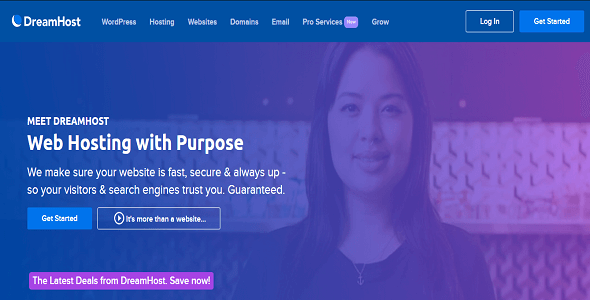This is a detailed caption for the described image:

---

The image is a horizontally oriented rectangular banner from the DreamHost website. At the top, a navy blue strip spans horizontally from left to right, featuring white font text and elements. On the left side of this strip, there's a logo that partially resembles a crescent moon in white, with the remainder of the moon filled in a brighter blue than the background. To the right of the logo, "DreamHost" is written in bold white font with the "D" and "H" capitalized, yet combined into a single word.

Adjacent to this, the menu items are listed in white font: "WordPress," "Hosting," "Websites," "Domains," "Email," "Pro Services" (with a small purple box labeled "New"), and "Grow." On the far right, two buttons are visible; the "Login" button features white font on a navy background with a white border, while the "Get Started" button has white font on a bright blue background.

Dominating the center-right of the image is a photograph of a woman with long hair, visible up to her chest. There's a subtle haze effect over her figure. To the left of her, bold white text reads: "Meet DreamHost." Below, in subheadline font, it says, "Web Hosting with Purpose." Further down, in smaller font, it states: "We make sure your website is fast, secure, and always up. So your visitors and search engines trust you. Guaranteed."

Beneath this text, there are two buttons: the "Get Started" button reappears in its bright blue form, and next to it, a rectangular button says "It's More Than a Website" with a play icon indicating a video.

At the bottom of this section, on the left side, a purple horizontal rectangular box with white lettering announces: "The Latest Deals from DreamHost - Save Now."

---